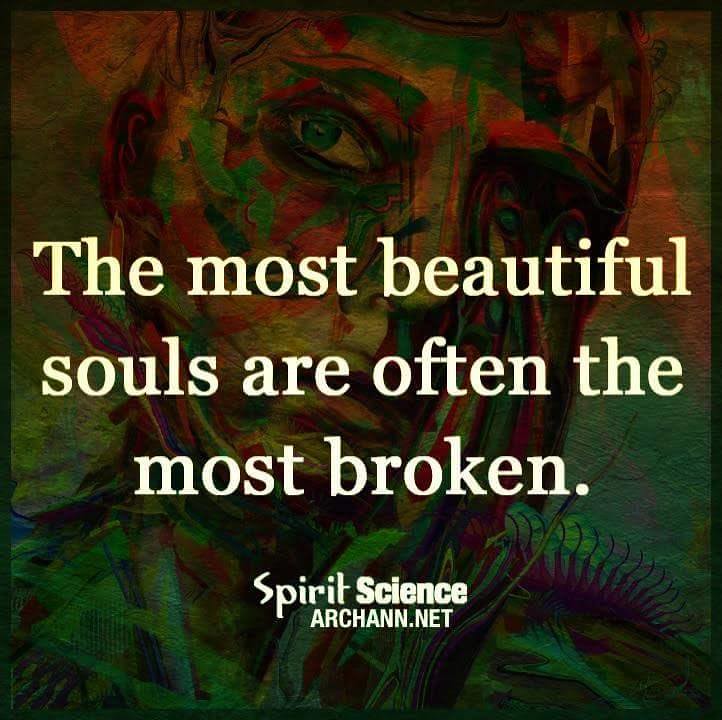The image is an abstract painting, which features a face that could belong to either a female or a male. The artwork is rendered in a variety of colors, predominantly green and red, with accents of yellow, purple, and orange, giving it an almost camouflage-like appearance. The face looks forward, one green irised eye visible while the other is covered by a hand. Superimposed on this multicolored background in large, white text is the inspirational quote: "The most beautiful souls are often the most broken." Below this, in smaller text, is the website "spiritsciencearchon.net."